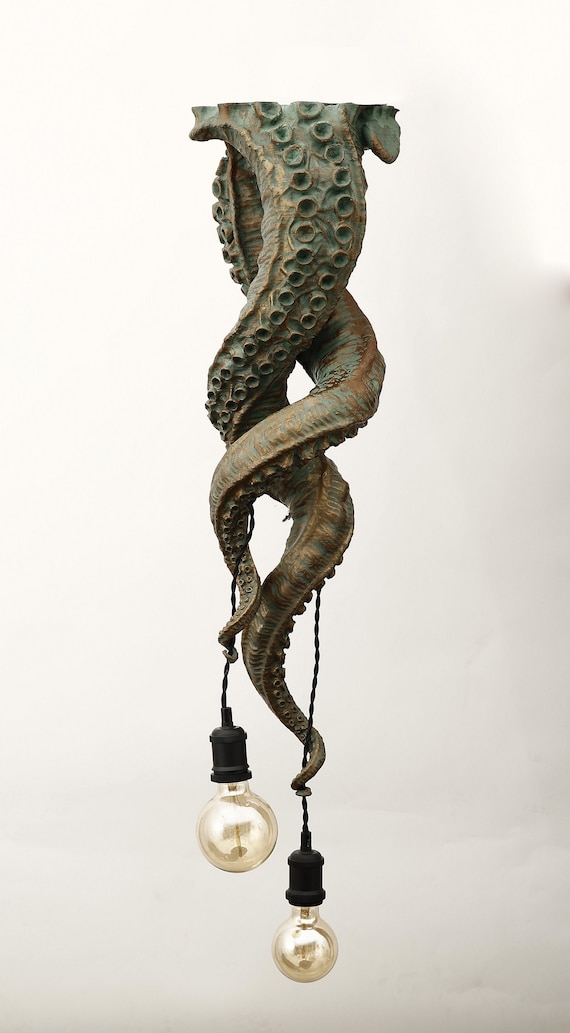The image depicts a realistic-looking sculpture set against a vertically oriented white, potentially beige, background, resembling a wall. The focal point of the piece is a pair of intricately crafted tentacles, possibly mimicking those of an octopus. These tentacles, appearing to be made from a material that resembles rusted and patinated bronze or copper with a greenish-brown hue, intricately wrap around each other, creating a dynamic, twisting shape. Each tentacle is adorned with detailed suction cups, enhancing the lifelike quality of the sculpture. From the bottom of the tentacles, two light bulbs are suspended. These bulbs, which have a pearl-like appearance, hang from simplistic black cords, adding a functional yet artistic element to the piece. The overall effect is that of a striking, nature-inspired light fixture, blending organic forms with industrial materials.